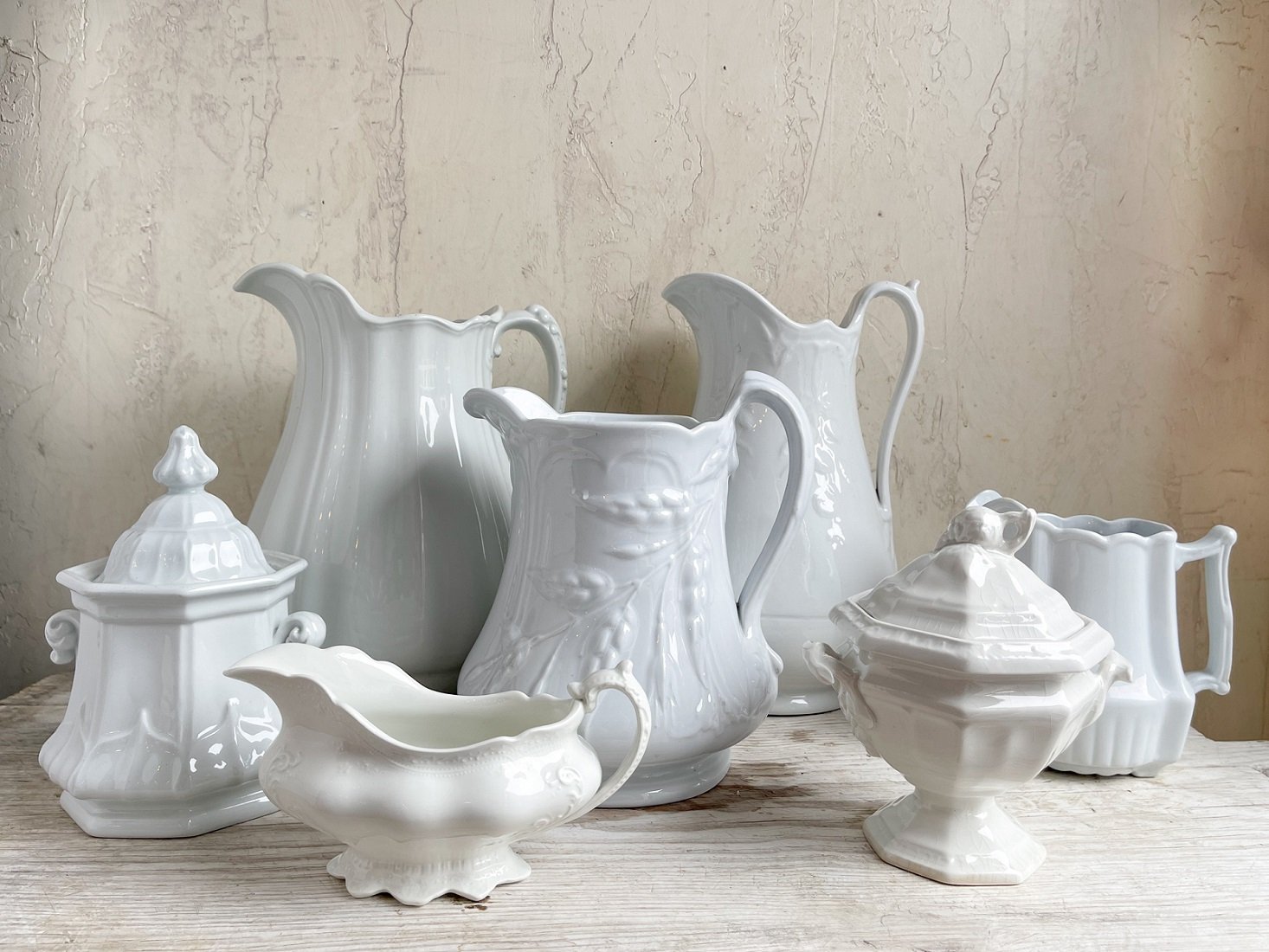The image is a detailed color photograph of an elegant china set arranged on a pale wooden table. The backdrop is a textured, off-white or cream-colored wall, giving a rustic and cozy atmosphere. In the foreground, there is an ornate gravy boat and a variety of cups, many with domed lids. Among these items, some appear to be sugar and flour dishes. The three tall pitchers, which are handle-right and lidless, are positioned at the back. These porcelain pieces are predominantly white, with some ranging to off-white or light blue, and adorned with intricate designs showcasing motifs of grains, grapes, and floral patterns. Each piece stands out for its unique pattern, contributing to the overall sophisticated and charming aesthetic.